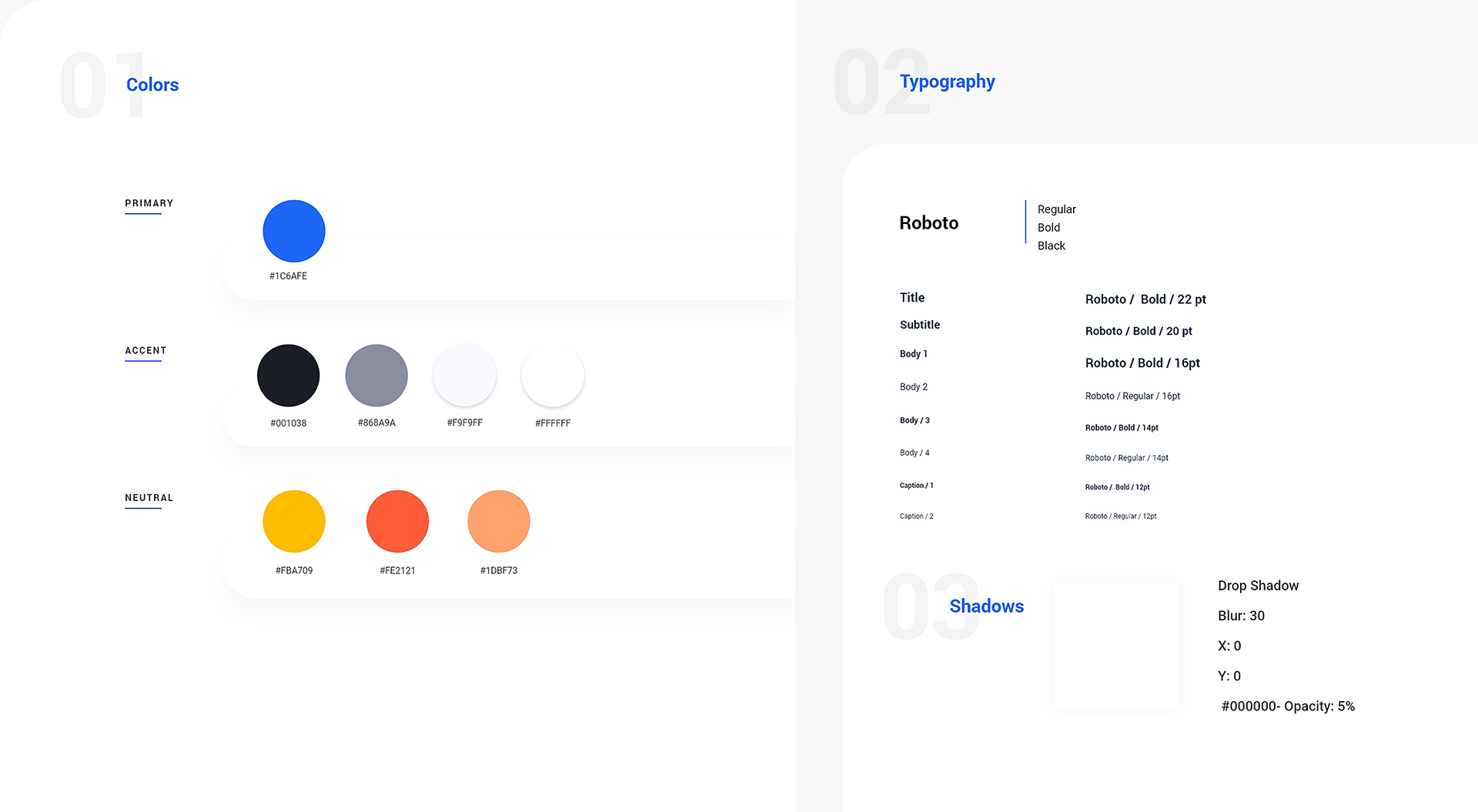**Image Caption: Comprehensive Design Elements Display**

The image presents a detailed layout of design elements, including colors and typography. 

**Left Side: Colors**
- **Primary Color:** 
  - A circle filled with royal blue, labeled "Primary," and accompanied by a small numerical identifier beneath it. 
- **Accent Colors:**
  - Four circles showcasing accent colors: Black, Gray, Very Light Gray, and White.
- **Neutral Colors:**
  - Three circles displaying neutral tones: Yellow, Red, and Orange.

**Right Side: Typography**
- **Font Family: Roboto**
  - Examples of different font weights: Regular, Bold, and Black.
- **Title:**
  - Displayed as "Roboto / Bold / 22pt."
- **Subtitle:**
  - Shown as "Roboto Bold 20pt."
- **Body Text:**
  - Four variations labeled Body 1 through Body 4:
    - Roboto Regular 16pt
    - Roboto Regular 14pt
- **Captions:**
  - Small text examples labeled Caption 1 and 2:
    - Roboto Bold 12pt

**Additional Design Element:**
- **Shadows:**
  - Description of drop shadow properties within a clear box:
    - Blur: 30
    - X: 0
    - Y: 0
    - Opacity: 5%

This image serves as a comprehensive guide to the essential design elements, including the specified colors and typographic styles, as well as their respective usages.